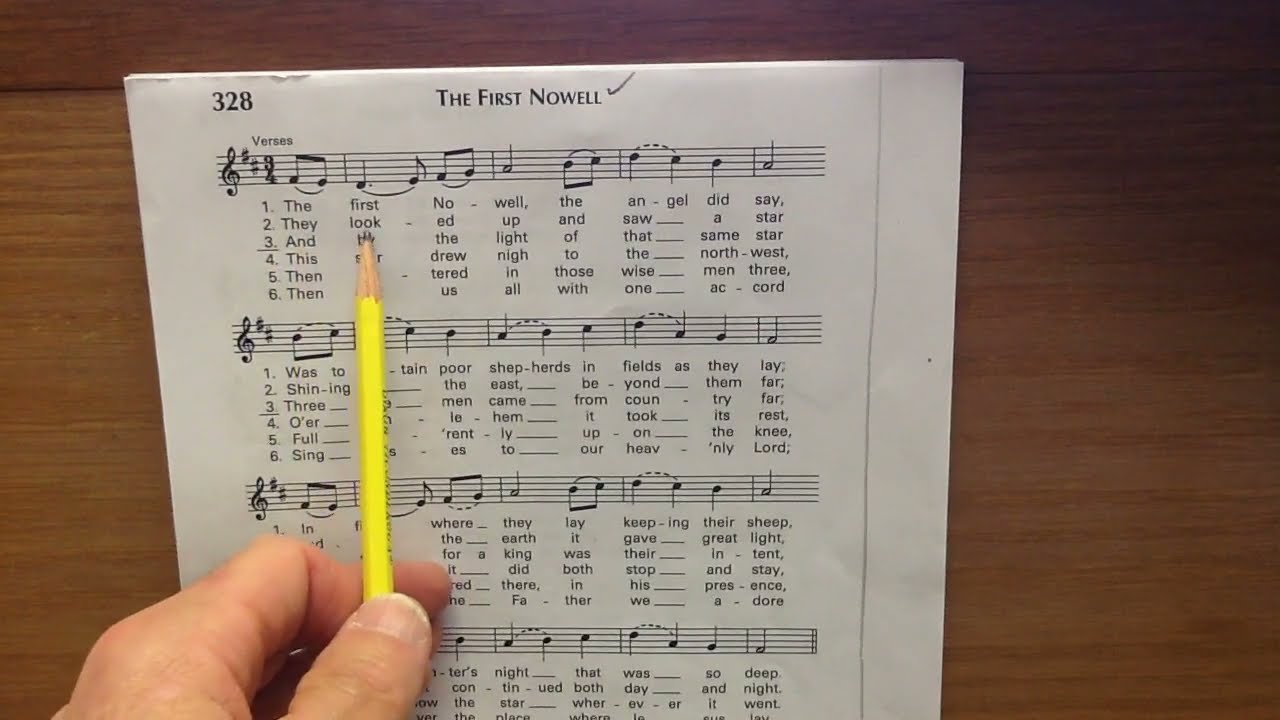The image depicts a close-up of a page from a music book resting on a medium-colored wooden table. The music sheet belongs to "The First Noel," spelled N-O-W-E-L-L, with the page number 328 printed in the top left corner. Below the title, the sheet features four stanzas, each starting with a treble clef, labeled as verses. Each stanza is accompanied by six lines of lyrics. The visible lines of lyrics include "The first Noel the angel did say," and "they looked up and saw a star." A Caucasian hand, whose thumb and index finger are visible, holds a bright yellow pencil. The pencil is pointing to the word "look" in the second line of the first stanza.